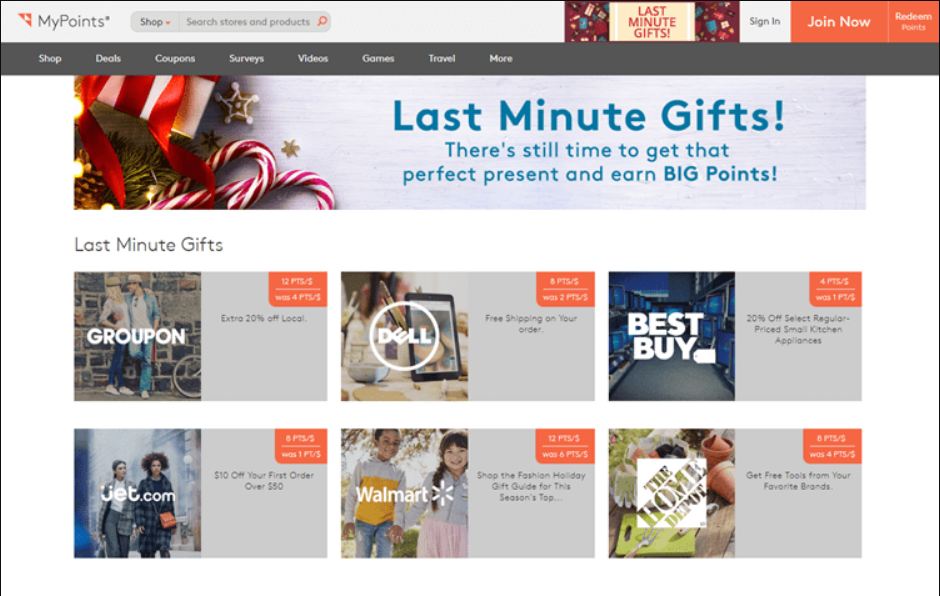This webpage from MyPoints prominently features the MyPoints logo with its distinctive triangle symbol at the top left corner. Adjacent to it, on the right, is a search bar labeled "Shop." Just below, a banner announces "Last-Minute Gifts" with vibrant images of festive decorations like candy canes, red ribbons, a white gift box, greenery, and pine cones, evoking a Christmas theme. The banner text is in blue, stating, "There's still time to get that perfect present and earn big points."

On the navigation bar beneath, various options are listed: Shop, Deals, Coupons, Surveys, Videos, Games, Travel, and more. Below that, the page reiterates the "Last-Minute Gifts" in a gray rectangle box stretching almost the full width of the page.

Further down, the page showcases six rectangular boxes with promotional offers. Each box is divided into two sections: the left features an associated photograph with the brand's name, and the right details the specific offer. For example:
- The first box displays "Groupon" with a photograph and an offer of an extra 20% off local deals.
- The additional boxes feature brands such as Dell, Best Buy, The Home Depot, Walmart, and Jet.com, each with their respective offers, earning points details, and points required for redemption. Though some details appear blurry, the offers clearly aim to attract users with enticing last-minute holiday deals.